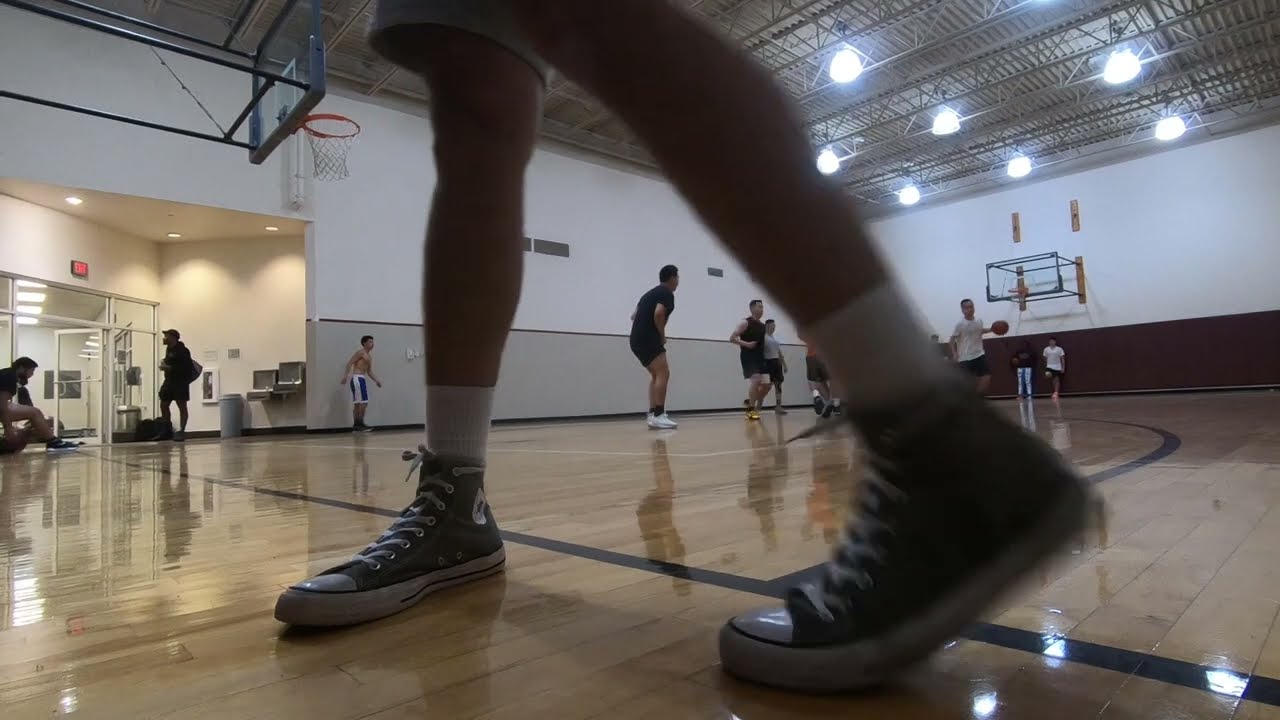In this horizontally aligned rectangular image of an indoor basketball court, the gym features white walls with a gray border on one and a brown border on the other. Wood flooring with black markings for out-of-bounds, free throw lines, and the three-point line adds to the court's typical appearance. Basketball goals are visible at both ends of the court, where several players are engaged in a game in the background.

The foreground prominently displays a person's feet, adorned in gray Converse high-top sneakers and white crew socks. Their skinny bare legs extend up to blurred shorts, suggesting movement. The left foot appears somewhat blurry. To the left in the background, the glass entry door with an exit sign above reveals someone sitting down and another person walking out. Near the gray wall, a man stands shirtless in striped blue and white shorts, likely watching the ongoing game. The gym’s shiny tan floors glisten, reflecting the light, and further in the distance, a water fountain can be spotted.